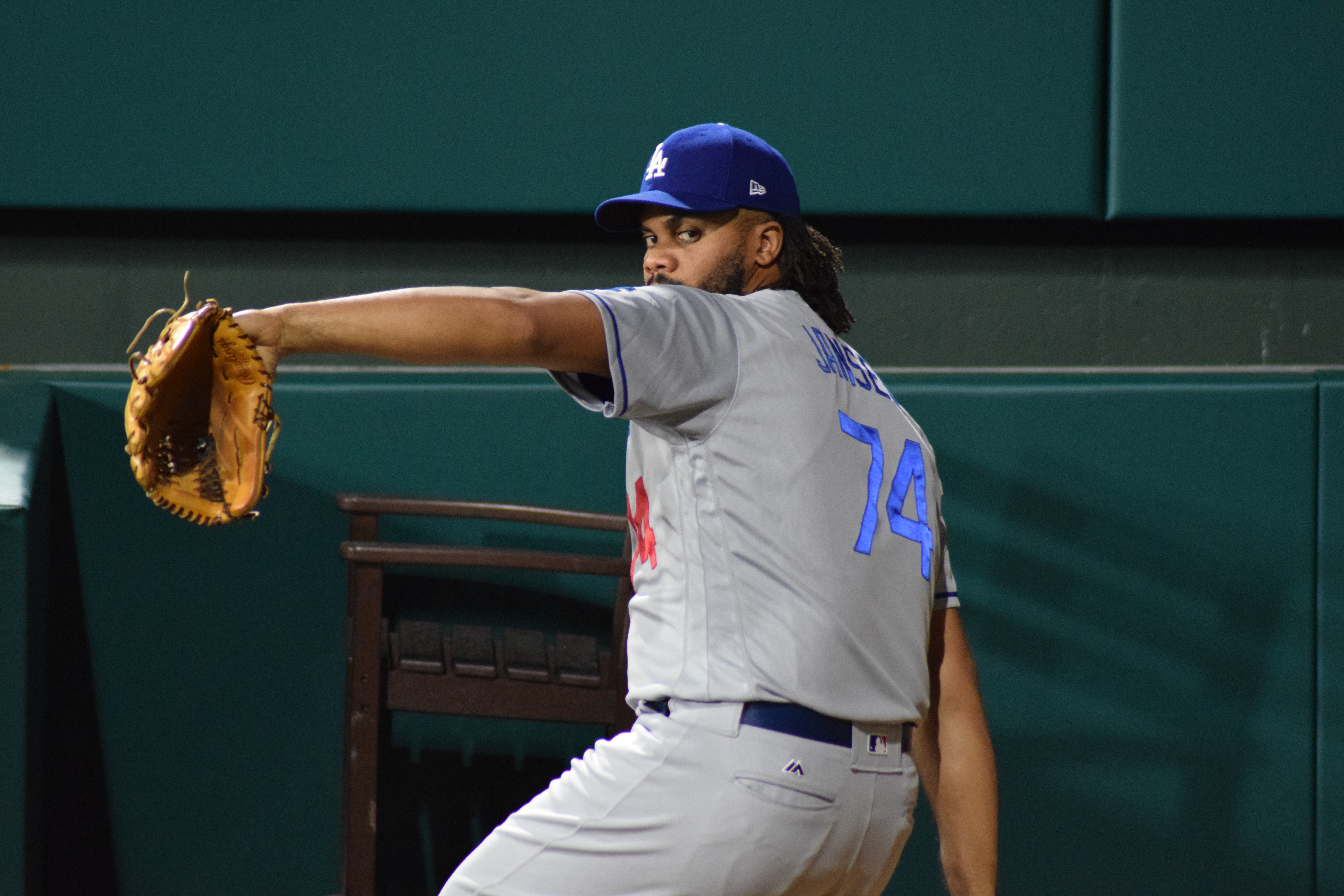A focused baseball player, wearing a gray uniform and a black belt, is warming up to pitch. He stands against a backdrop of a green padded wall, extending his left arm outward, revealing the inside of his glove. His right hand, although out of the frame, hangs by his side, poised to throw the ball. He wears a dark blue baseball cap adorned with white "LA" lettering and has a serious expression as he gazes straight ahead. The back of his jersey displays blue letters and the number 74, identifying him as Jensen. There is some red lettering on the front of his jersey, though it is not visible in the image.